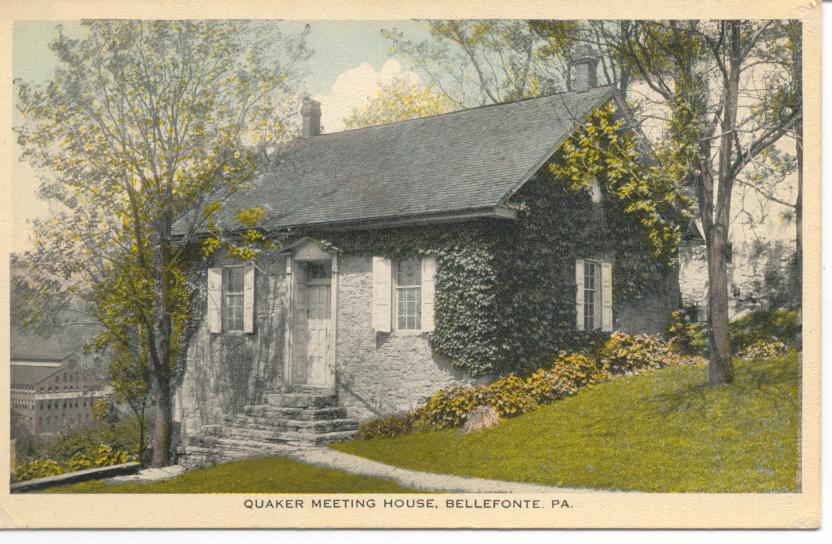The image appears to be a vintage postcard featuring a historic Quaker Meeting House located in Belafonte, Pennsylvania. The central subject is a one-story brick and wood house with ivy climbing one side. The house sports white shutters on its windows and a prominent A-frame gabled roof. The front features a white door with a glass window, accessible via a set of five stone steps leading down to a walkway and a well-kept, though not vibrant, green lawn. This scene is set against a sky with blue and white clouds, and is framed by two young trees with autumnal leaves.

Although the house itself is presented in black and white, elements like the grass, the sky, and the foliage have been colorized, giving the impression that the building is part of an older photograph embedded in a more contemporary, colorful landscape. The front view, along with a partial side view showcasing additional windows and the ivy, captures the house from a three-quarter angle. The photograph is bordered by a beige frame, adding to its vintage postcard feel. In the background, additional buildings can be seen down the slope to the left. At the bottom of the postcard, the caption reads, "Quaker Meeting House, Belafonte, PA."